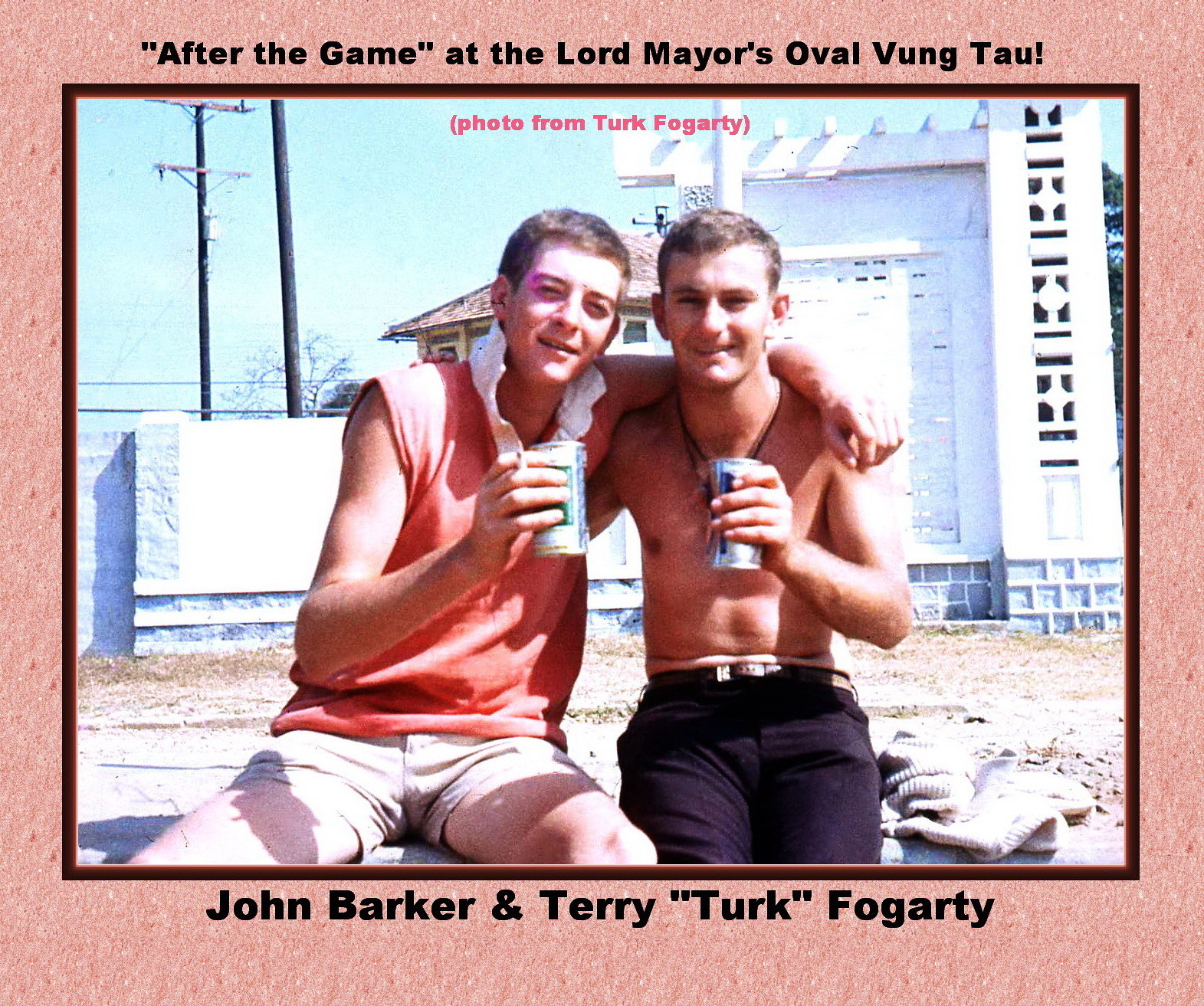This photograph, set in Vietnam at the Lord Mayor's Oval Vung Tau, captures two young men sitting together on what appears to be a concrete edge or bench, possibly at the edge of a hill. Both men are holding cans that look like beer. The man on the left is wearing a short-sleeved orange tank top with a white collar and light-colored shorts, and has his arm around the man on the right, who is shirtless but dressed in black trousers with a black belt and a necklace. The man on the right also has his arm around his companion. Behind them stands a white building or buildings and a long white stone or concrete wall, as well as some power lines. The sky appears blue, suggesting a clear day. The photograph has a peach-colored border with black text at the top reading, "After the game at the Lord Mayor's Oval Vung Tau," and at the bottom, "John Barker and Terry Turk Fogarty." Additionally, red text on the photo itself reads, "Photo by Turk Fogarty." Both men are white with short brown hair.